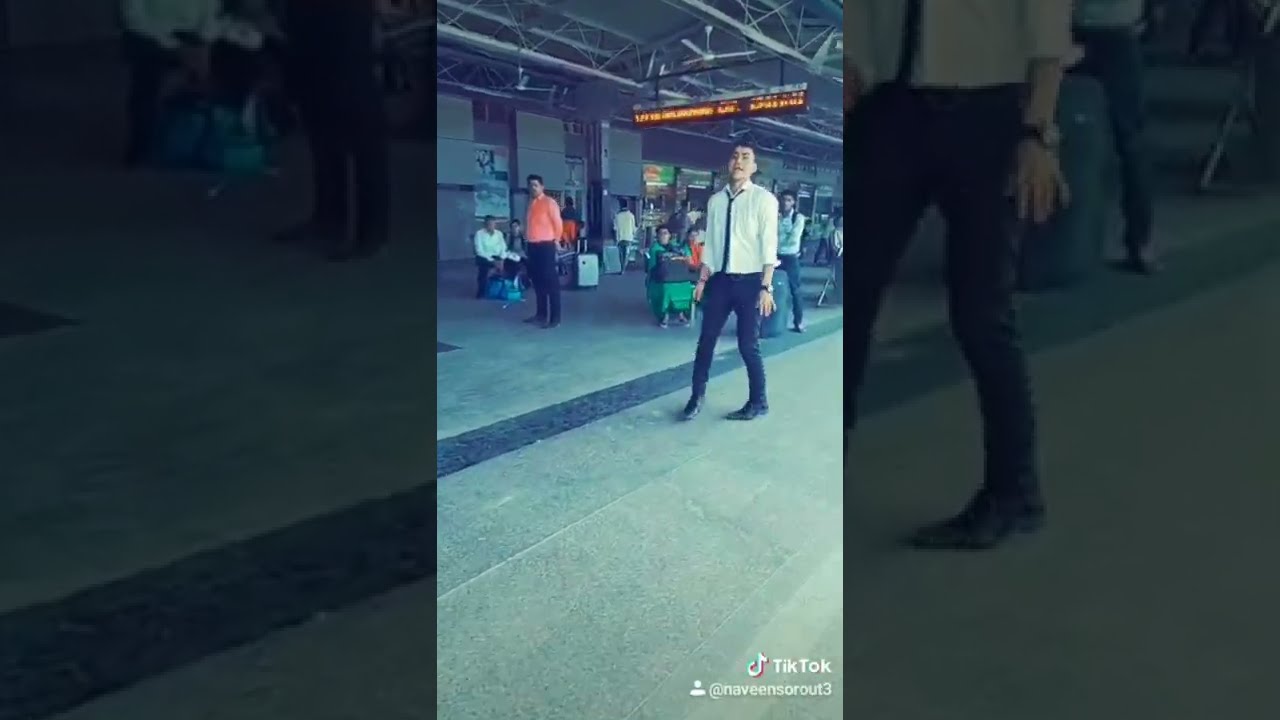The horizontal rectangular TikTok image is divided into three sections: left, center, and right. The central and primary section features a slightly grainy, out-of-focus scene taken outdoors during the daytime, likely at a train station or terminal. The focal point is a man dressed in a long-sleeve white button-down shirt, black tie, black pants, and dress shoes. He stands with his arms stiffly at his sides and his feet positioned oddly apart, giving him a peculiar stance. His mouth is open, adding to his unusual pose. Behind him, various people are either sitting or standing, some appearing as if they're waiting with luggage. A woman in a green dress with a black bag in her lap is seated, while another man in black pants and an orange shirt is seen to the left. In the distant background, lit-up signs and windows, likely from shops, can be seen.

On the image's lower right corner, the TikTok logo and handle, "@NaveenSorout3," are visible. The left and right sections of the image are close-ups that are blurred and darkened. The left side shows a person's legs and part of the sidewalk, while the right side showcases the man's pants and shirt up to his chest, revealing he is wearing a watch on his left hand. The entire scene is framed by high ceilings and steel beams, with a possible black strip on the floor indicating areas to stand, adding to the train station ambiance.